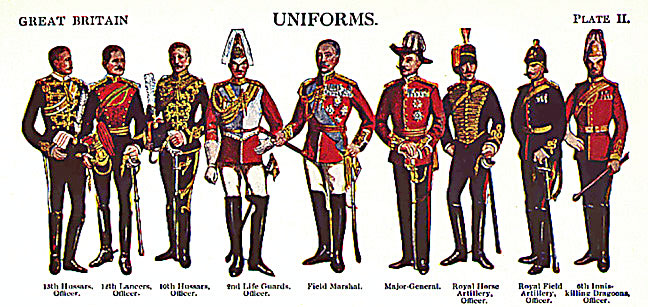This detailed image captures a hand-drawn poster of British soldiers, each adorned in different military uniforms. Displayed prominently across the top are the words "Great Britain". In the center, the text reads "Uniforms," while the top right corner is marked with "Plate 2". The poster features nine men standing side by side, each wearing distinctive uniforms that represent various ranks and regiments.

Each soldier's attire is meticulously detailed with an emphasis on black boots worn by all. Their coats predominantly come in red and black, with a few yellow accents such as roping. Additionally, two soldiers wear white pants, and a major general sports long pants with red stripes. Each man holds a sword, adding to the military aesthetic.

The soldiers are shown in varied poses, looking in different directions, which creates a dynamic array. Labels beneath each figure specify their roles: the leftmost figures include the "13th Hussars Officer," "12th Lancers Officer," and "10th Hussars Officer." In the center are higher ranks such as the "Field Marshal" and "Major General." Continuing right, the labels indicate "Royal Horse Artillery Officer," "Royal Field Artillery Officer," and finally, what appears to be the "6th Inniskilling Dragoons Officer."

This poster serves as an illustrative display of the diverse and elaborate uniforms worn by British officers, capturing a snapshot of military history through detailed and colorful artistry.